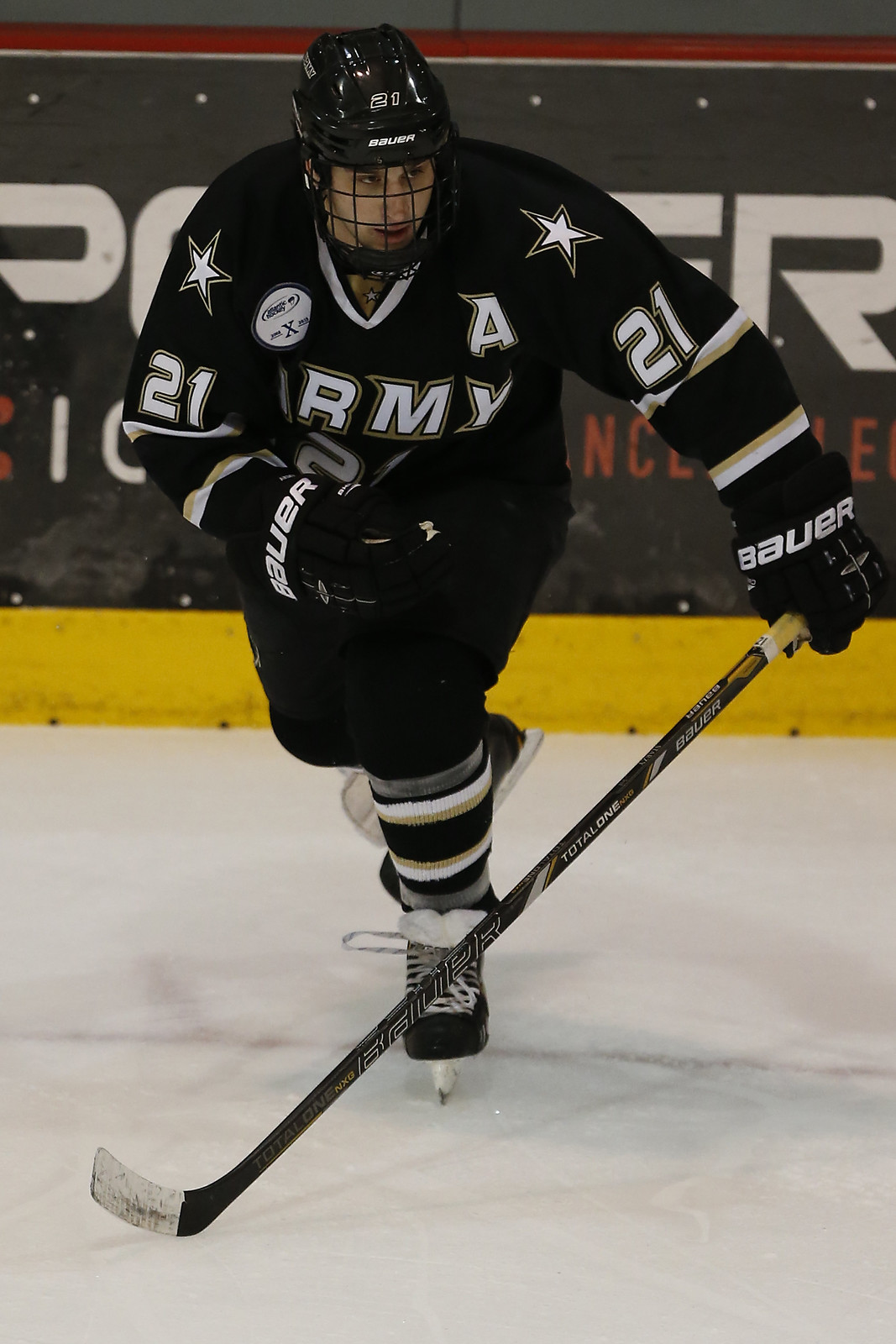This detailed color photograph captures a hockey player in action on an ice rink. The player, skating forward and facing the camera, is clad in a black and white jersey with the word "ARMY" partially visible, and the number 21 prominently displayed on the front, as well as on both sleeves. Adorning the top of his sleeves are white stars, signifying his role as an alternate captain, indicated by the letter 'A' on his jersey. The player also sports black Bauer gloves, black pants, and white, black, and yellow striped socks. His black skates feature white laces.

The hockey player's black helmet, which includes protective face caging, also bears the number 21 and the Bauer brand in white lettering. He is holding a Bauer Total 1 NXG hockey stick in his right hand. The stick, decorated in black, white, and yellow with the player's number 21 and the brand name multiple times, is topped with white tape wrapped around the head. The background features an advertisement on the rink's boards, though the complete text is obscured by the player. The wall behind has a black background with hints of white and red lettering, and a yellow strip at the bottom and a red strip at the top, all set against the ice surface of the rink.